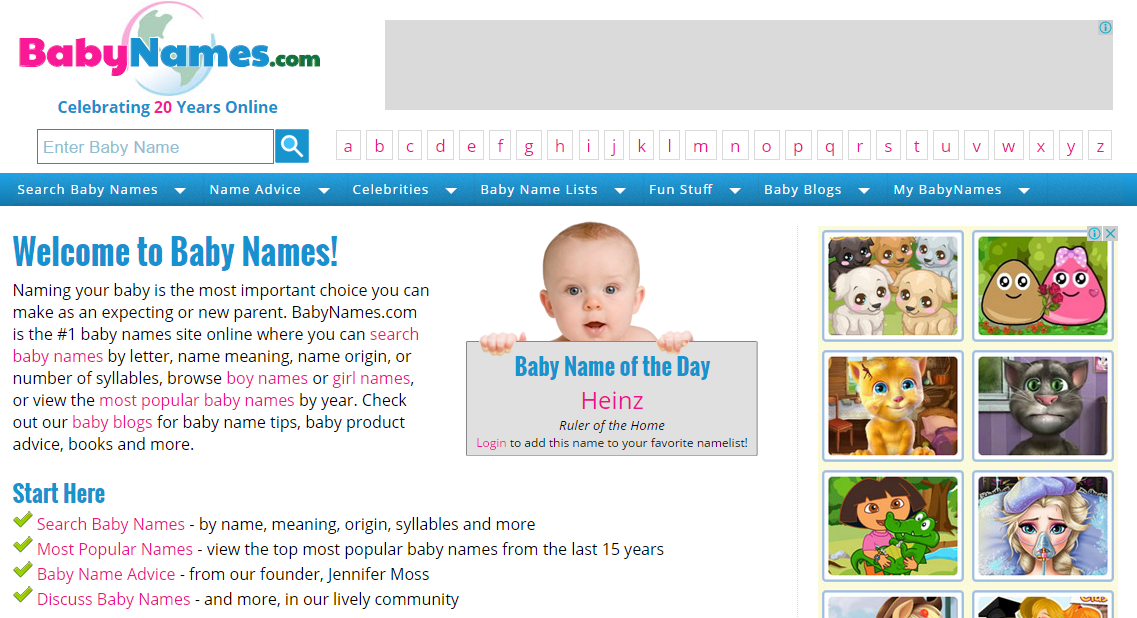This image features the homepage of the website BabyNames.com. The page sports a clean white background. In the upper left corner, the BabyNames.com logo is prominently displayed; the logo consists of a globe, with the word "Baby" written in pink, "Names" in blue, and ".com" in green. Below the logo, it proudly states "Celebrating 20 Years Online."

Prominently positioned, there is a search box prompting users to "Enter a Baby Name" with a corresponding search button for easy access. To the right of the search box, there is a gray-colored placeholder, presumably for an advertisement. Beneath this, an alphabetically arranged set of letters from A to Z allows users to easily browse baby names by their starting letter.

Following this section, a blue navigation bar provides links to various site features including "Search Baby Names," "Name Advice," "Celebrities," "Baby Name List," "Fun Stuff," "Baby Blogs," and "My Baby Names." Each of these options features drop-down menus or icons that suggest further subcategories.

Below the navigation bar, welcoming text introduces the BabyNames.com site. A call-to-action labeled "Start Here" lists multiple starting points for new visitors. At the center of the homepage is an image of a baby, which adds a touch of charm to the interface. Just below this image, a gray box highlights the "Baby Name of the Day," which, in this case, is "Hines." To the right of this featured name, a few cartoon characters add a whimsical and friendly element to the site's overall appearance.